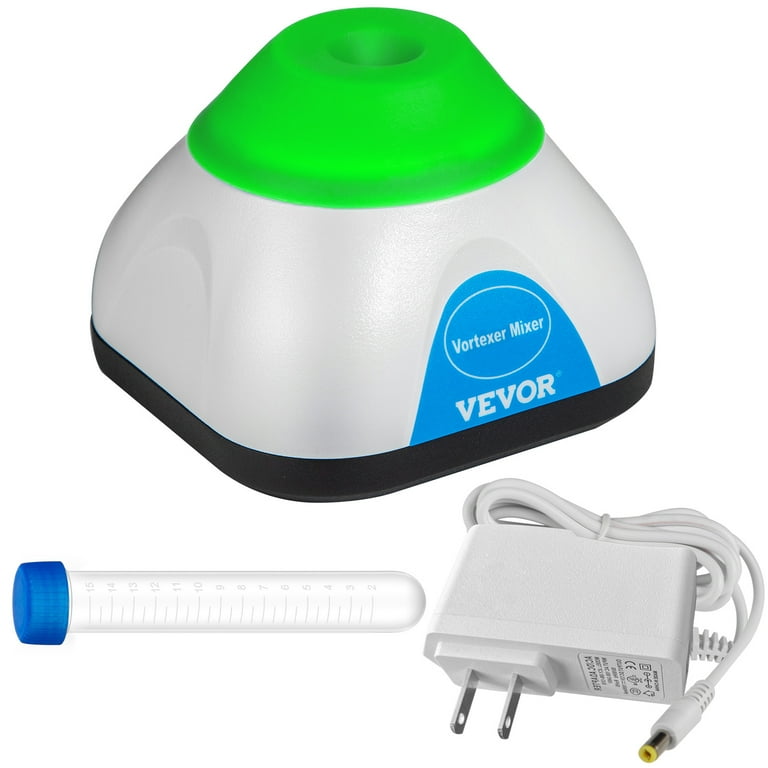This is an up-close image of a contemporary Vortexer Mixer by VEVOR. The mixer itself has a pyramid-shaped design with a neon lime-green hollowed-out cylindrical top, presumably for inserting a test tube. The body of the mixer is white with a centered blue triangular label reading "Vortexer Mixer" in white text, followed by the brand name "VEVOR" beneath it. The base is black, providing a sleek contrast to the lighter colors above. The image also includes a test tube with a blue cap, likely intended for use with the mixer, and an electrical adapter with a wound cord, highlighting its requirement for a power source. The equipment appears to be intended for laboratory use, and the clean white background and focused composition suggest this is a catalog shot designed to showcase the mixer and its components effectively.